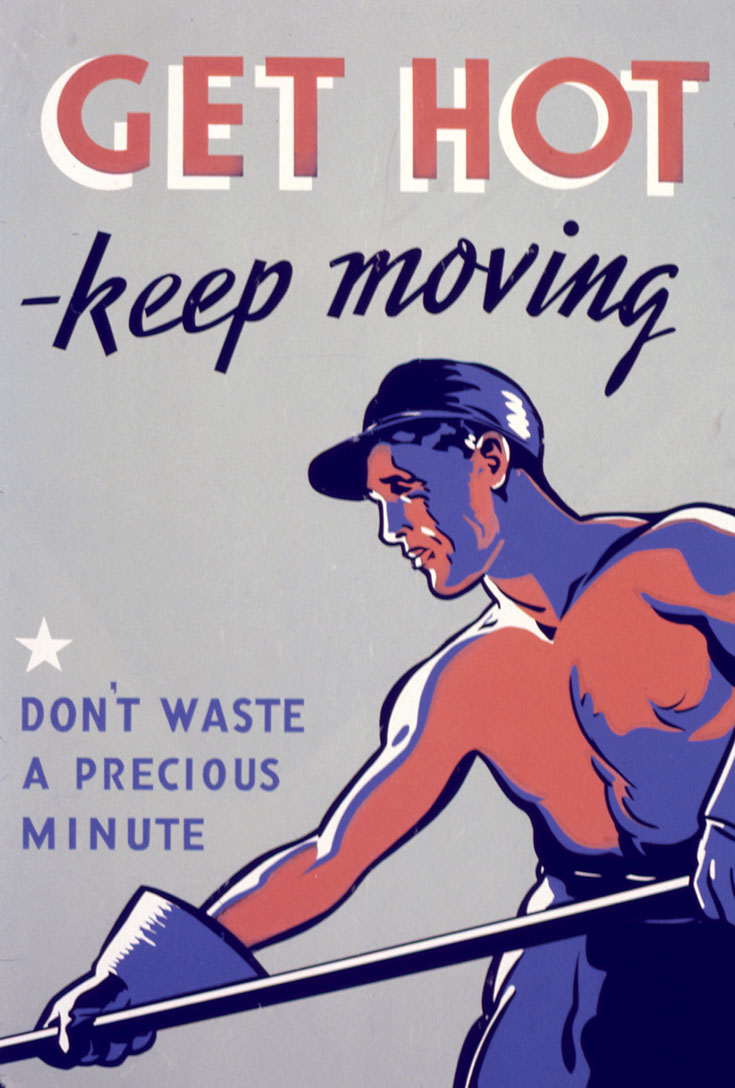This poster, set against a gray background, features a striking illustration of a muscular, shirtless man engaged in outdoor labor. He is depicted in vibrant red and blue tones, with his chest painted red and much of the rest of his body, including his face, neck, and pants, in shades of blue. He wears a distinctive blue hard hat and blue gloves, which resemble rubber gloves typically used for washing dishes. In his hand, he grasps a long, black pole that could be a mop, broom, shovel, or rake. 

The text on the poster delivers a motivational message: "GET HOT" is prominently displayed at the top in bold, red, all-caps letters with a white outline. Below it, "Keep Moving" is written in black. Near the man’s torso, a small white star punctuates the space above the phrase "Don't Waste a Precious Minute," which is rendered in the same blue as his painted body parts. Overall, the poster's dynamic composition and vivid colors emphasize the importance of perseverance and continual effort.